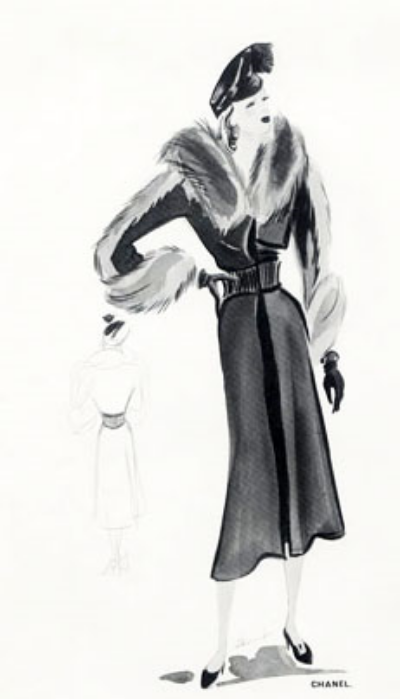This image is a vintage Chanel advertisement sketched in black and white on an off-white background. At the center, it features a detailed charcoal drawing of a high-status woman, reminiscent of the 1940s or 1950s. She is adorned in an elegant ensemble, comprising a luxurious fur coat with plush fur trim around the collar and sleeves. The coat, which extends into a slender dress-like form, accentuates her waist and hips, possibly cinched with a belt. She wears striking black high heels and dark lipstick, adding to her sophisticated aura. Atop her head rests a plumy black hat. A faint outline of a mannequin, showcasing the same outfit, is lightly sketched to the left of her. Below, in the bottom right corner, the luxury brand name “Chanel” is inscribed in black text, cementing the image as an advertisement for the illustrious fashion house.